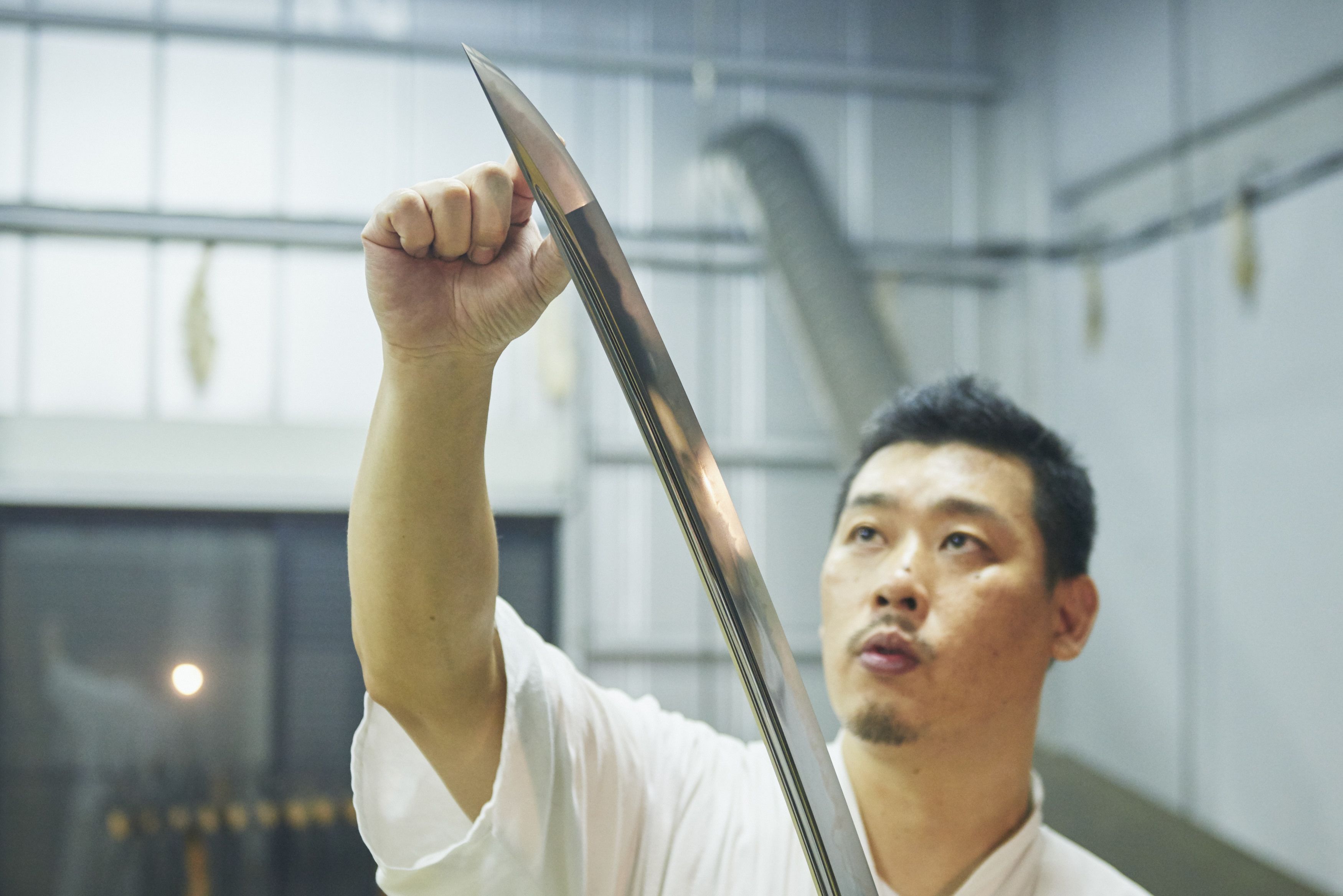The photograph features an Asian man who appears to be either a sushi chef or a professional swordsman, wearing a white, short-sleeved top reminiscent of attire commonly seen in sushi restaurants. He has short black hair and a goatee. The man is carefully examining a long, powerful, and shiny silver sword with a dark groove along one edge. Holding the sword in his left hand, which is out of the frame, he delicately touches near the tip of the blade with the index finger and thumb of his right hand and looks intently at it. The background reveals a setting with white, factory-like walls, interspersed with metal beams or pipes, and a dark window on the left reflecting both the man and the camera flash. Additionally, there is a yellow circle on the wall, and a glass double door positioned towards the lower left of the frame. The light source appears to be coming from the upper left corner of the room.